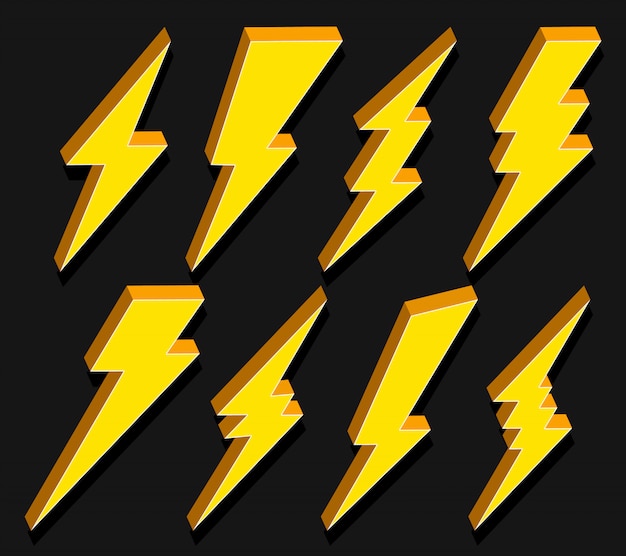The image features a dark gray, almost black background, overlaid with two rows of stylized lightning bolts—four on the top row and four on the bottom. Each lightning bolt is yellow, with a thin white outline around its edge. Adding to the depth, these bolts have a 3D effect: the left sides of the bolts are shaded a light brown, while the tops and right sides are shaded a warm tan. A drop shadow in dark gray or nearly black further enhances the three-dimensional appearance. These eight bolts, all exhibited in slightly different shapes and variations, resemble classic depictions of electric bolts or stylized icons you might find in logos or t-shirt designs.